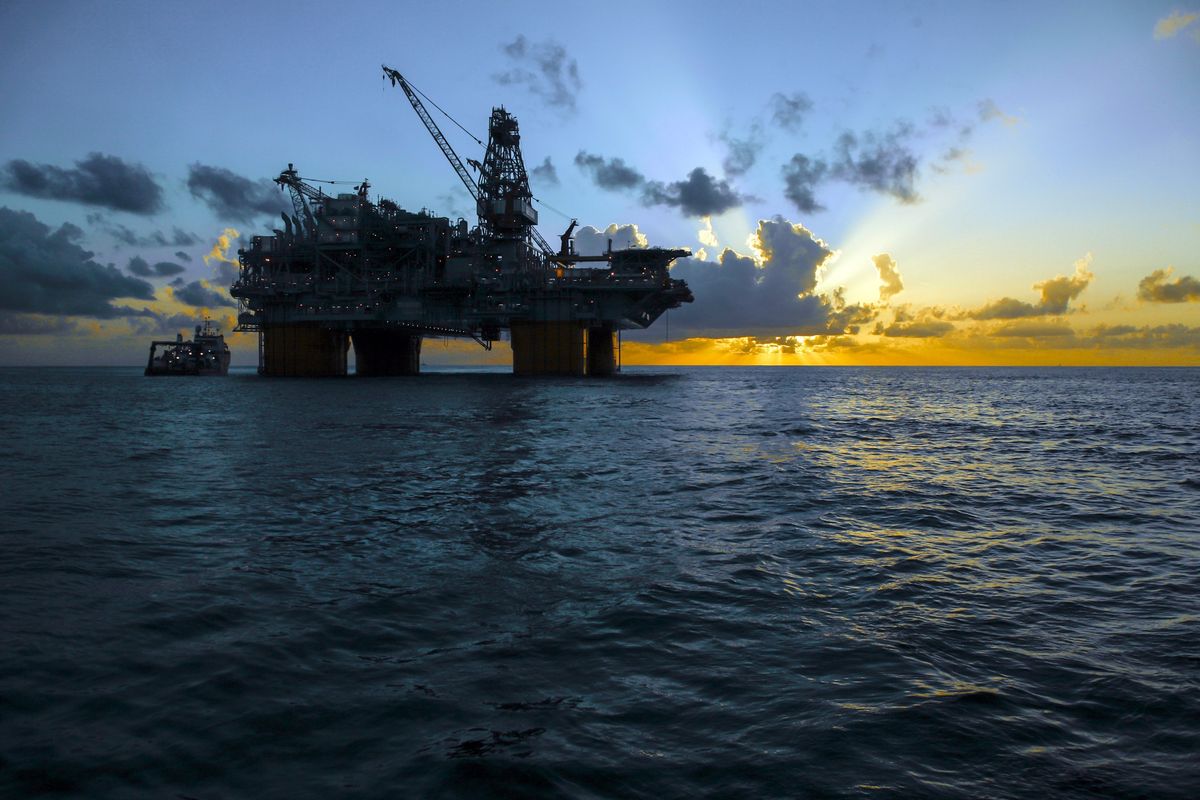In this photograph, an imposing oil rig dominates the left-hand side of the scene, set against the deep blue expanse of the ocean. The rig, with its towering structure elevated above the water on sturdy pillars, is equipped with a large crane and a smaller crane. Adjacent to the rig, a diminutive supply or refueling boat sits in the water, highlighting the massive scale of the oil platform. The ocean waves, gentle and calm, mirror the tranquility of the scene. The sky, occupying the upper half of the image, transitions from a pale blue to a golden hue as the sun sets, casting a warm yellowish-orange glow. Scattered clouds partially obscure the sun, softening the light and adding texture to the sky. The overall composition captures the serene yet industrious atmosphere of this oceanic landscape at dusk.